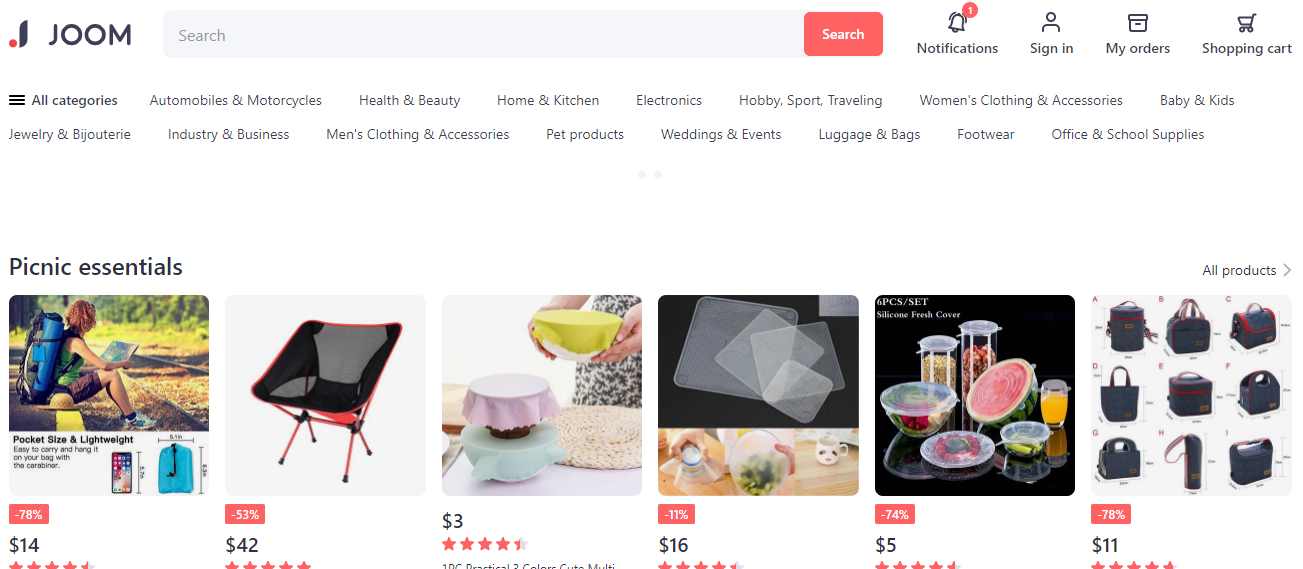This image is taken from the Joom shopping website, displaying a clean, white background. In the top-left corner, the website name, "JOOM," is prominently visible in bold letters. To the right, there is a user-friendly search bar accompanied by a red search button. Notifications are indicated by a bell icon with one alert, followed by options for "Sign In," "My Orders," and "Shopping Cart."

Below this section is a horizontal menu listing various categories such as "All Categories," "Automobiles and Motorcycles," "Health and Beauty," "Home and Kitchen," "Electronics," "Footwear," and "Office Supplies." Towards the far right, a special category titled "Picnic Essentials" is highlighted. This section features several items available for purchase, including a pocket-sized, lightweight cell phone holder, a portable chair, flexible coverings for bowls, and a versatile cooler bag. Each product is showcased with an image, making it easy for users to browse and select items for their needs.